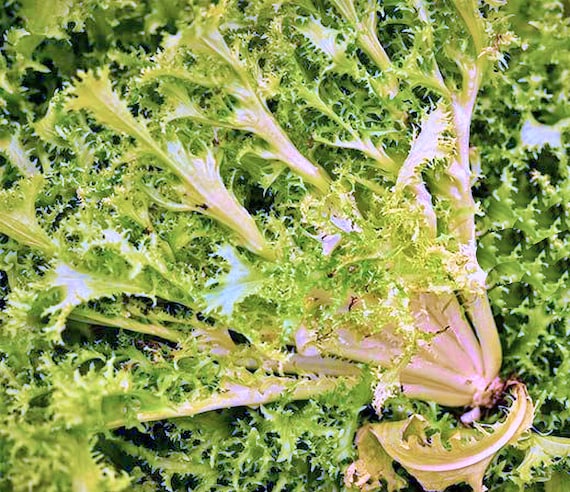This up-close photograph captures a detailed view of frisée lettuce, showcasing its intricate texture and unique form. In the background, a bed of frisée leaves sets the stage, while prominently in the foreground, a cluster of frisée leaves is arranged horizontally. The image clearly displays the area where the roots have been cut, transitioning into stalks that burst outward with robust, curly leaves. The distinctive curls and edges of the frisée emphasize its characteristically bitter, yet visually appealing nature. The arrangement of the frisée is positioned diagonally across the frame, adding a dynamic element to the composition.